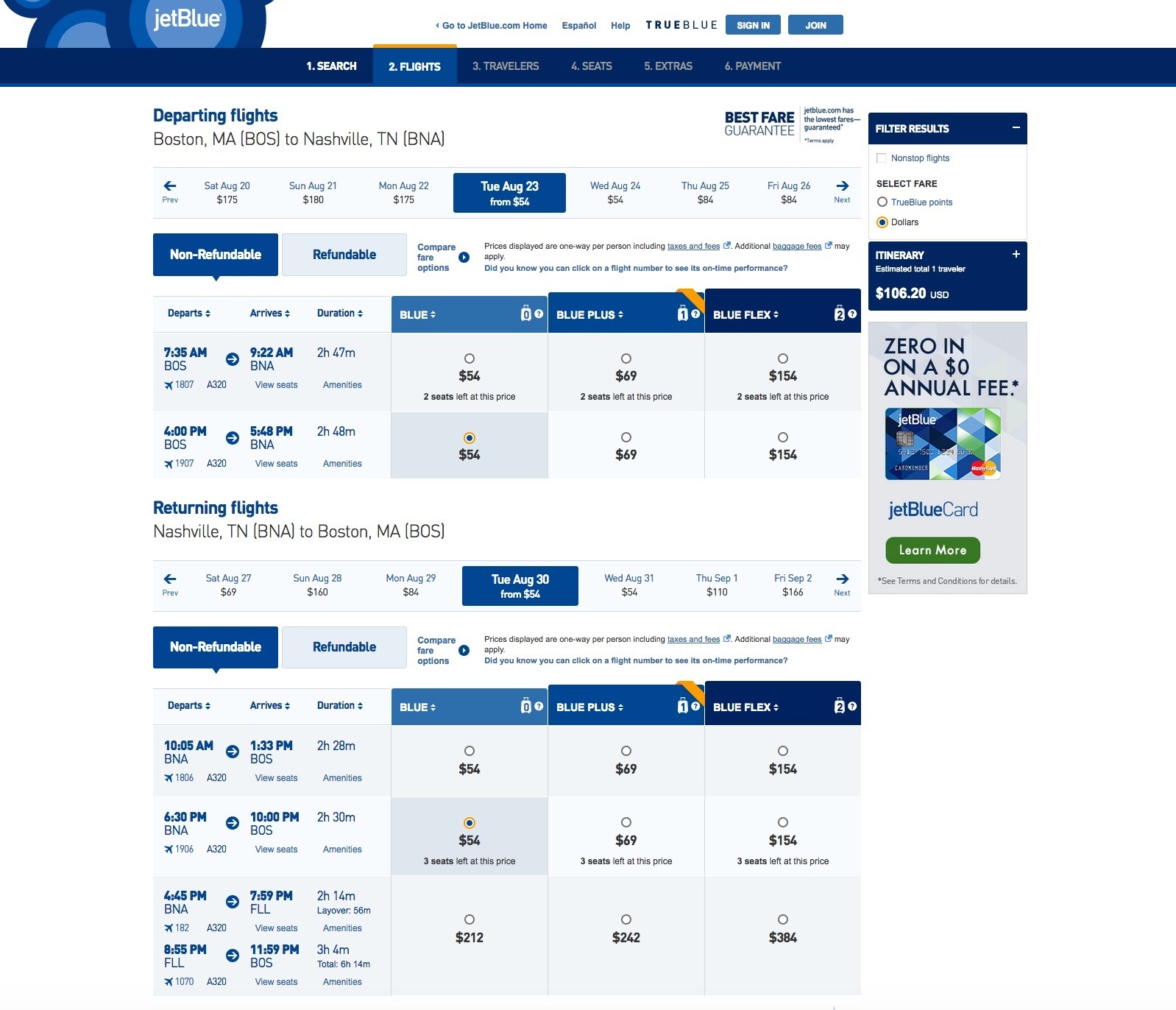This image captures the front page of JetBlue's website, prominently showcasing their TrueBlue rewards program on the right side. The left side features a blue graphic consisting of two interlocked circles with a flat element on top. At the top right corner, there are options to sign-in and log in.

Beneath this section, a dark blue horizontal line spans across, dividing the webpage into different sections labeled: "Search," "Flights," "Travelers," "Seats," "Extras," and "Payments." 

Further down, the webpage provides information on departing flights, specifically from Boston, Maine to Nashville, Tennessee, including detailed flight information. On the right side, there's an option to filter results, possibly by fare, though the text is somewhat difficult to decipher. 

The main content features departure details with non-refundable taglines, listing fare options such as Blue, Blue Plus, Blue Flex, among others. An itinerary is highlighted with a price of $106.20. Additionally, there's a promotion for a JetBlue credit card spotlighting a $0 annual fee, with a call-to-action button in a green bar to "Learn More."